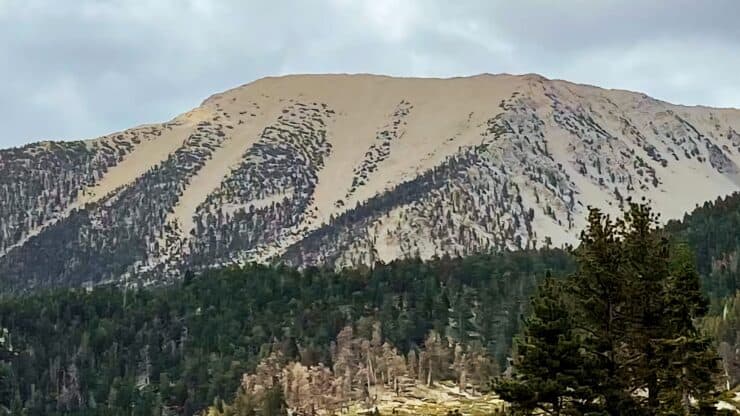The image captures a majestic snowy mountain under a dark overcast sky, with a landscape rich in various types of trees. The mountain’s peak is rather flat, with a gradual slope on the left and a less steep slope on the right that maintains an extended ridgeline. Although the mountain is mostly covered in snow, patches of brown and tan earth, as well as small black rock formations, are visible, appearing like shadows but actually being sections of dense forest. Amidst the greenery, sporadically dotted dead trees can be seen, more prevalent towards the left-hand side of the forest. The bottom center of the image is notably lit by sunlight, illuminating a smaller section of dead trees and grassy terrain with warm brown and tan hues. The foreground is dominated by an abundant forest of tall, vibrant green pine trees, accentuating the lushness of the surrounding landscape despite the cloudy, overcast conditions above.